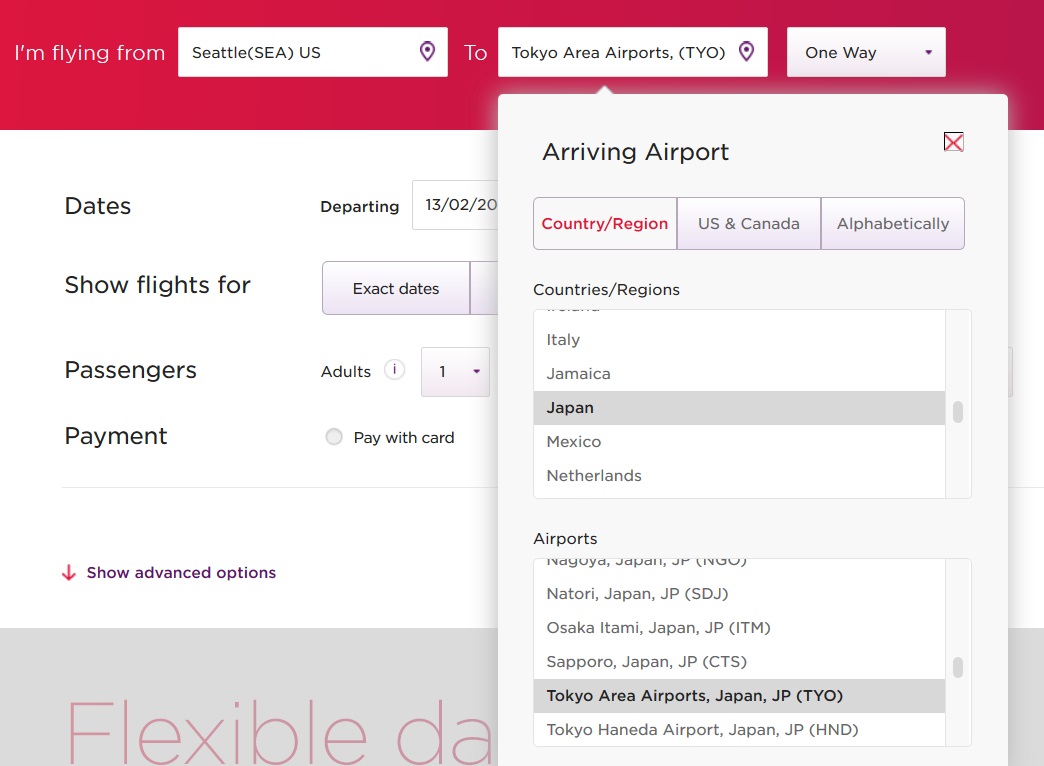The image features an interface for flight booking. At the top, there's a red header with the text "I'm flying from" next to a white input box labeled "Seattle, SEA [US]" with a location pin icon on the right. Below it, the text "To" appears next to another white input box labeled "Tokyo Area Airports, TYO."

From the "Tokyo Area Airports" box, a drop-down menu opens, presenting a larger white box with "Arriving Airport" at the top right corner, accompanied by an "X" icon to close the menu. Below this, there are three selectable buttons labeled "Country/Region," "U.S. and Canada," and "Alphabetically" on the far right. 

Further down, a list with a scroll bar shows "Country/Region" options, including Italy, Jamaica, Japan, Mexico, and the Netherlands. Beneath this scrollable country list is another heading, "Airport," followed by additional options: Nitori, Japan; Osaka; Atami, Japan; Sapporo, Japan; Tokyo Area Airport, Japan; and Tokyo Narita Airport, Japan.